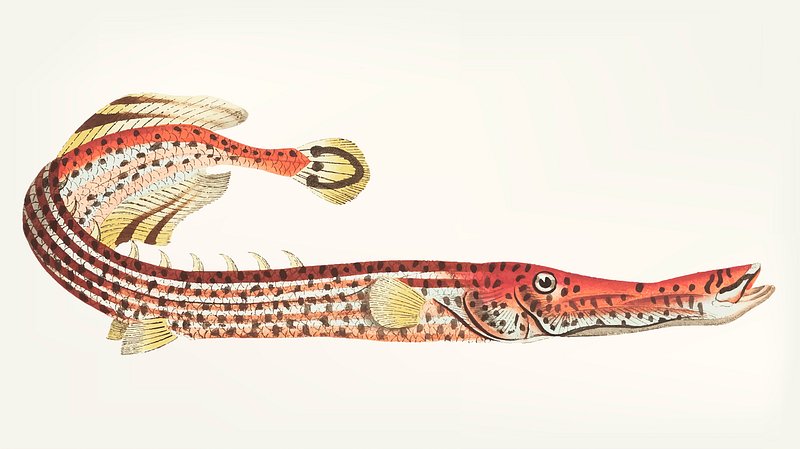This is a detailed digital watercolor illustration of a peculiar, elongated fish that closely resembles an eel. The image displays the creature curling in a serpentine motion, occupying the central portion of an off-white background. Its face, positioned on the right side of the composition, features a long, snouted mouth and round white eyes with black pupils. The body extends leftward before looping back towards the top center, causing the tail fin to sit just above and behind the head.

The top of the fish is painted in a striking reddish-orange or rust copper hue, adorned with small black spots and squiggly lines, particularly on the snout. The underside and flanks exhibit a lighter copper tone, peppered with additional black dots. Highlighting its aquatic nature, the fins on its back are tan with delicate feather-shaped brown stripes, while the fins near its gills and the tail fin shimmer in a golden yellow. Notably, the tail fin is detailed with a distinctive black horseshoe shape with a dot at its center. The overall visual effect conjures the sense of an ancient, possibly prehistoric marine creature, making it suitable for art sites or educational materials reminiscent of old textbook illustrations.